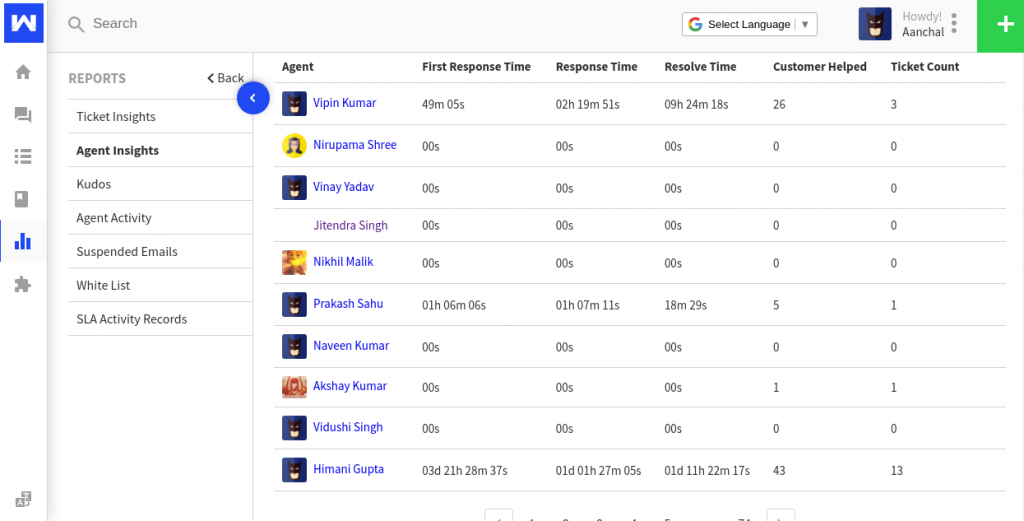The image displays a customer service software interface, likely designed for a customer support team, given the various monitoring tools and metrics presented. At the top, a search bar featuring the Google logo and a language selection option can be seen. Adjacent to the search bar, there's a greeting message, "Howdy Anchal," followed by several menu options: Agent Insights, Ticket Insights, Kudos, Agent Activity, Suspended Email, Whitelist, and SLA Activity Records.

The interface prominently features an agent list in the middle, showcasing detailed metrics for each support agent. The first agent listed is Vipin Kumar, with his statistics on first response time, overall response time, resolution time, the number of customers helped (26), and ticket count (3). Additional agents listed include Nirupama Shree, Vinay Yadav, Jintendra Singh, Nikul Malik, Prakash Sahu, Naveen Kumar, Ash A. Kumar, Vidushi Singh, and Himani Gupta. The same metrics are displayed for each agent, offering a comprehensive view of their performance.

The design of the interface is predominantly white, with subtle gray accents, presenting a clean and minimalistic appearance suitable for professional use. Judging by the names, the software may be utilized by a team based in India.